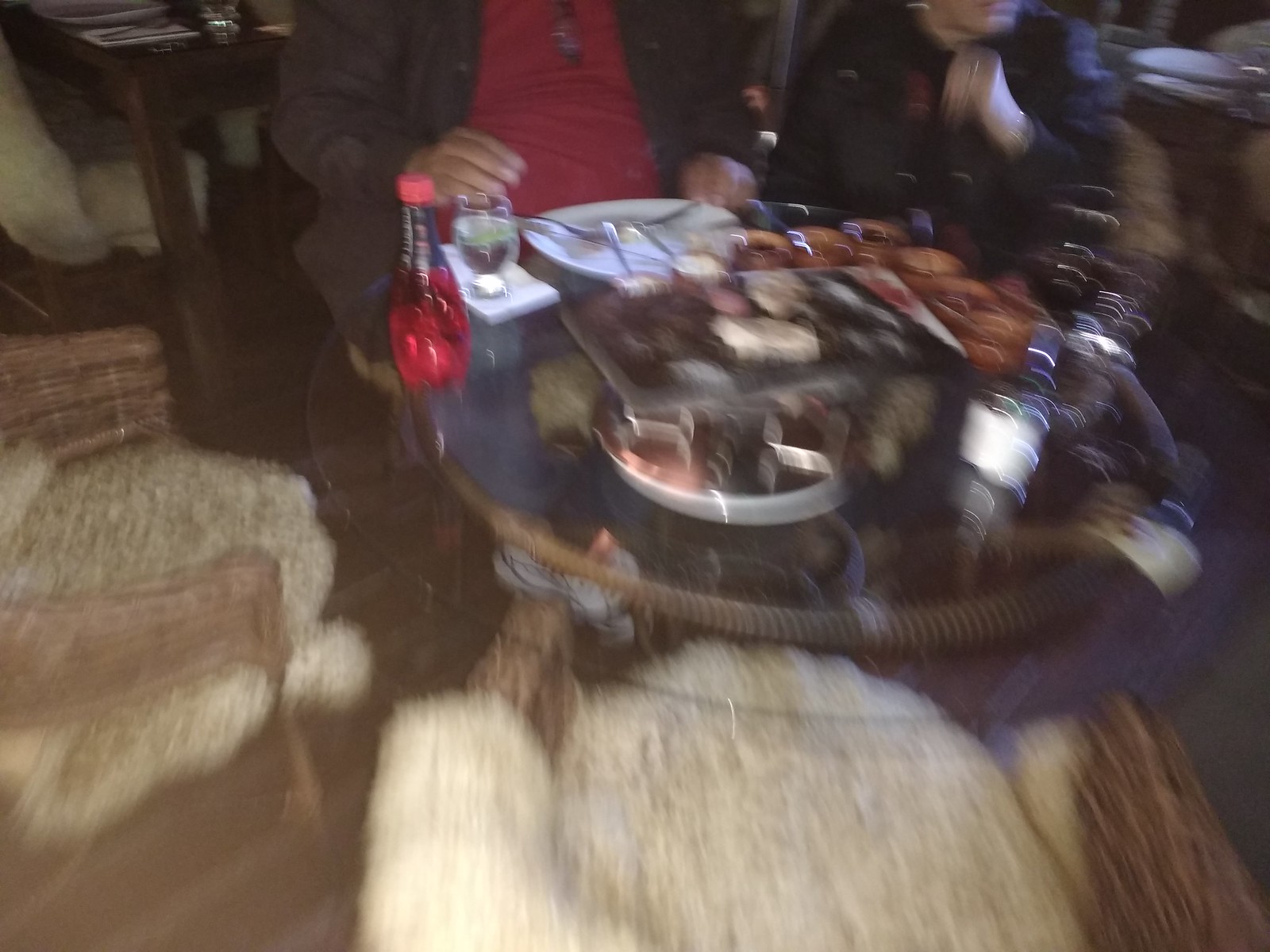The image depicts a round glass table set for a meal, surrounded by four chairs. Two of these chairs are empty, featuring wicker frames with cream-colored fabric cushions. The other two chairs are occupied by a man and a woman, though their faces are obscured due to the blurred effect in the image.

The man is seated in one of the chairs, wearing a red shirt and a brown jacket, with glasses hanging from his shirt. In front of him, there's a white plate with silverware, suggesting he has recently finished eating. Beside his plate, a glass containing what appears to be wine or a similar beverage is placed.

Next to him sits a woman in a black jacket. While details about her are indistinct due to the blur, you can see a platter of various foods in front of her. Additionally, there is a red-colored drink in a glass container on the table, which could be soda or wine.

The overall atmosphere of the image is somewhat blurred, giving it a dreamy and unfocused appearance, capturing a casual dining scene involving partial visibility of two individuals and their meal on the glass table amidst the empty wicker chairs.